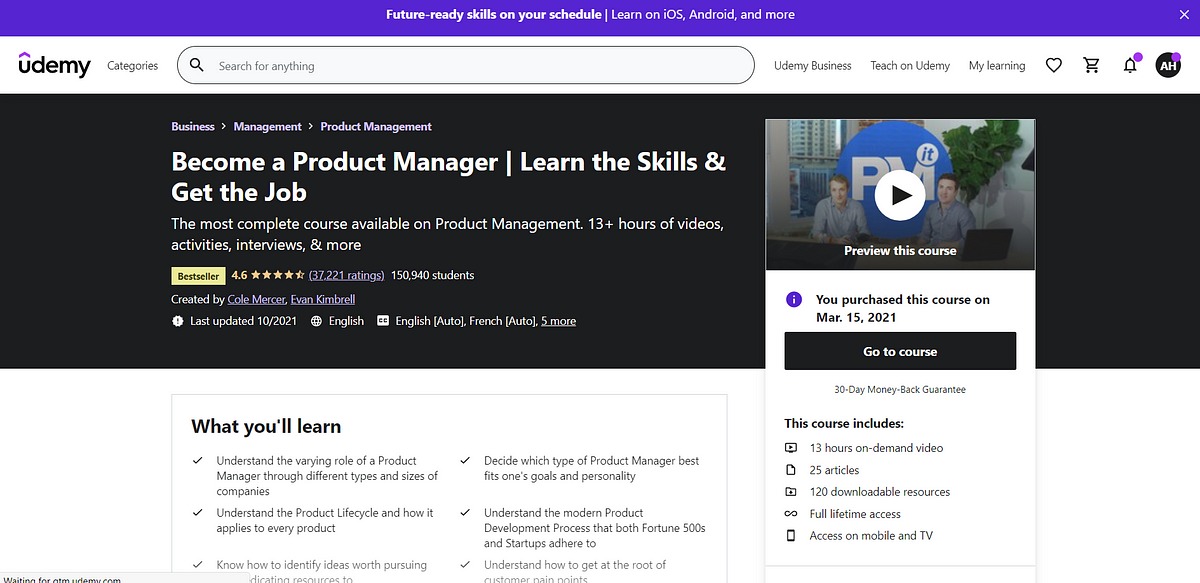Here is a detailed and cleaned-up caption for the given image:

---

This image is a screenshot from the Udemy website. At the very top of the page, a prominent purple bar displays the text "Future-ready skills on your schedule. Learn on iOS, Android, and more." Below this bar, the website header includes the Udemy logo, a navigation menu with categories, a search bar that says "Search for anything," and options for "Udemy Business," "Teach on Udemy," and "My Learning," followed by different icons.

Further down, a large black rectangular banner highlights a course titled "Business Management: Product Management." The banner states, "Become a Product Manager: Learn the skills and get the job. The most complete courses available on Product Management," featuring "13+ hours of videos, activities, interviews, and more." A yellow "Bestseller" badge accompanies a 4.6-star rating based on 37,221 reviews and 150,940 students. The course creators are Cole Mercer and Evan Kimbrell, and it was last updated in October 2021. The course is available in English, with auto-translated versions in French and five other languages. To the right, a pop-up window offers a preview of the course with a play button, noting "You purchased this course on March 15th, 2024." There's also a "Go to course" button within a black box and a "30-day money-back guarantee" label.

At the bottom left, another rectangular section titled "What you'll learn" lists various key takeaways from the course, each accompanied by a checkmark icon. 

---